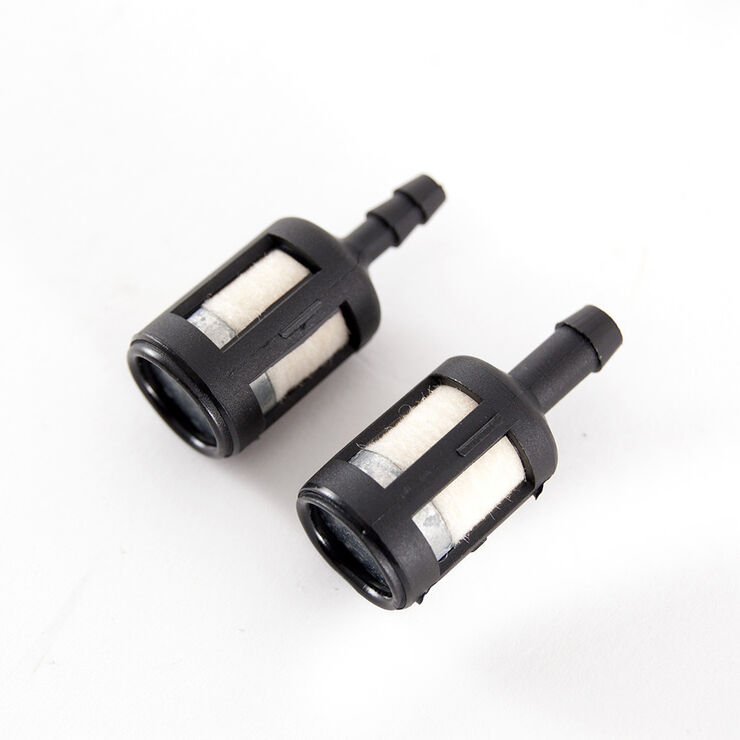The image features two black and white cylindrical objects positioned diagonally on a white background. Each object is predominantly black plastic with white components inside. They resemble cylindrical cans with elongated narrow tips extending from their sides. The cylinders have two rectangular openings on their bodies, exposing white, cottony filters inside. These openings correspond with a design that might suggest a light or a filter mechanism. The objects also have multiple prongs at their tips and a plastic earpiece-like attachment for comfort. The setting appears to be a plain white table or countertop, giving a neutral backdrop which highlights the detailed construction of the objects. The bottom of each cylinder features a rounded black lip. The objects could be elements from a machine, such as filters or valves, owing to their shape and openings, but their exact function remains unclear.